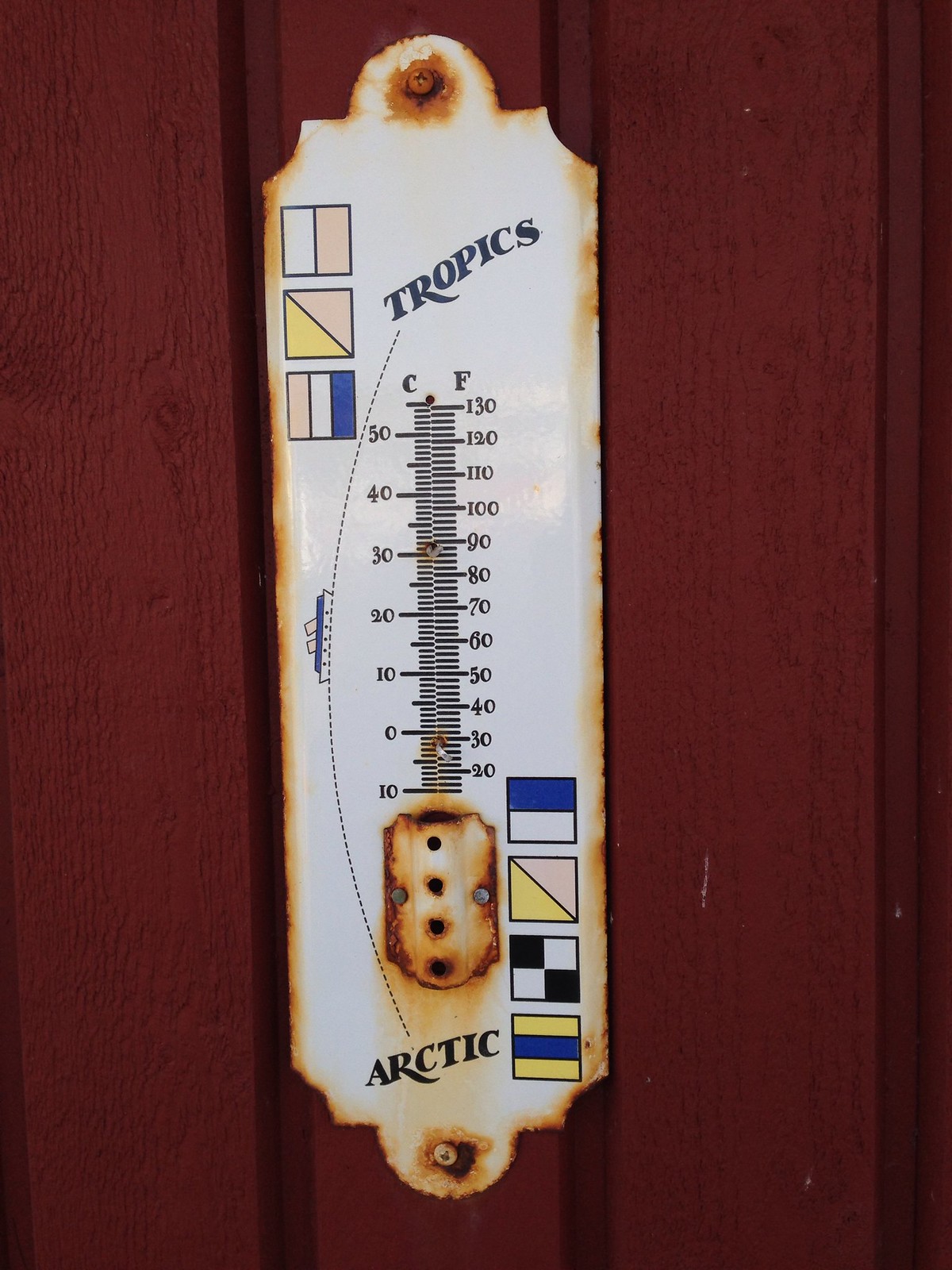A sophisticated, mercury-free thermostat is mounted on the wall, displaying the brand name "Tropics." Its sleek design and advanced features suggest superior functionality, ideal for efficiently regulating indoor temperatures. The device stands out against a predominantly cool-toned backdrop, highlighting its significance in providing precise climate control.